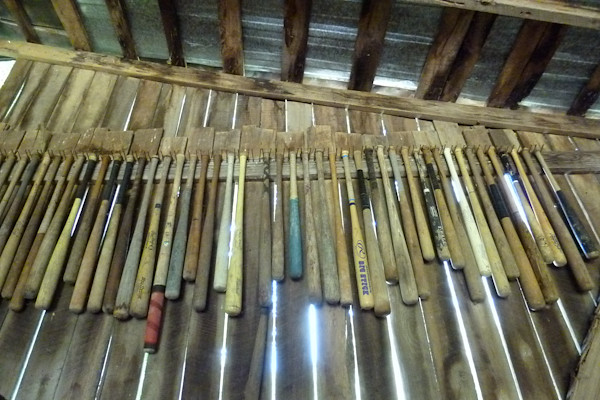The image depicts a collection of baseball bats hanging on a wooden plank, set against a rustic wooden wall. The bats vary in color and length, featuring plain light brown, turquoise blue, black, and a uniquely designed bat with a red-striped tip. The camera angle looks slightly upward, giving a sense of the bats being displayed on a shelf. The background is a wooden structure, possibly a shed, characterized by slanted roofing with metal sheets and planks that are not securely fastened, allowing light to seep through the gaps. The overall setting conveys a simple, DIY storage solution likely within a wooden building.